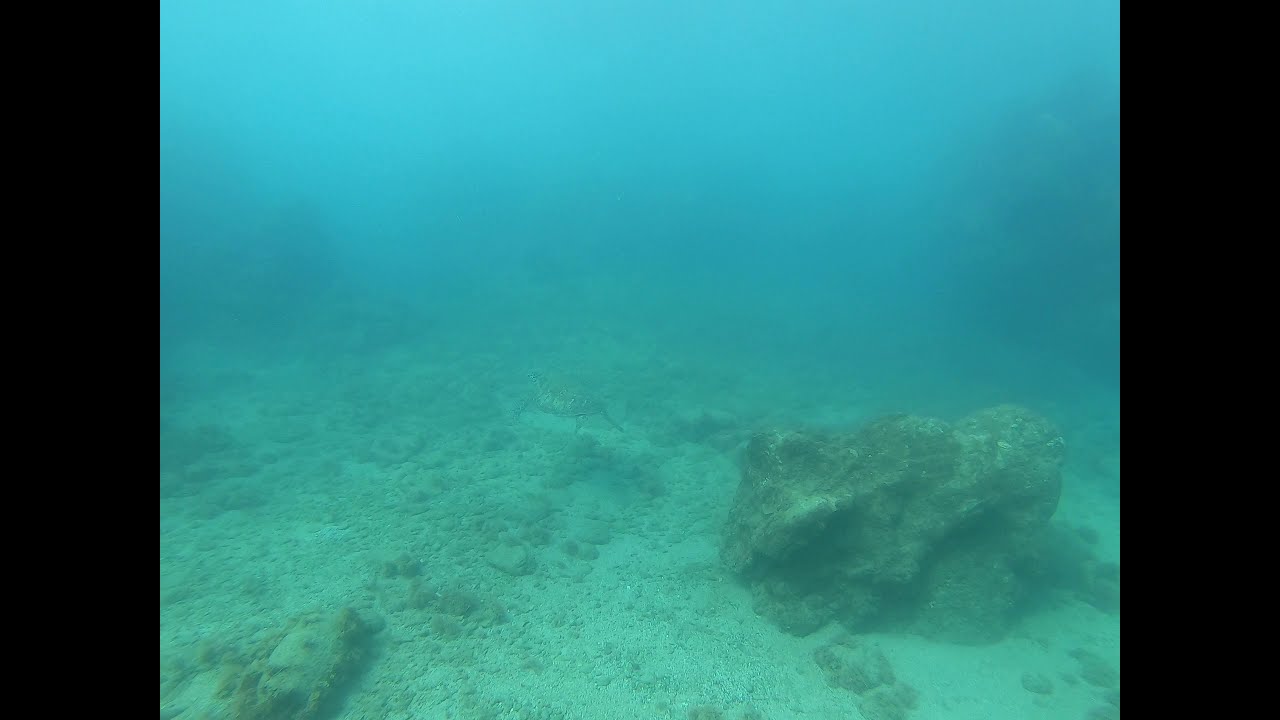This underwater photograph captures a murky, cloudy scene with a predominantly bluish-green tint. The image, taken at the bottom of a body of water, presents a sandy or gravelly seabed scattered with numerous small rocks and a few larger ones. Notable is a big rock towards the lower right corner, covered with what appears to be green moss or algae. The background is characterized by an ombre effect, transitioning from a darker blue at the top to a lighter turquoise as it descends, though visibility is poor due to the foggy, blurry water. The entire scene is framed by bands of black along the left and right edges. In the middle of the image, a somewhat indistinct object, possibly a seahorse or turtle, adds to the intrigue, though it remains unclear due to the haziness. No signs of fish or other marine life are evident, reinforcing the stillness and serenity of this underwater landscape.